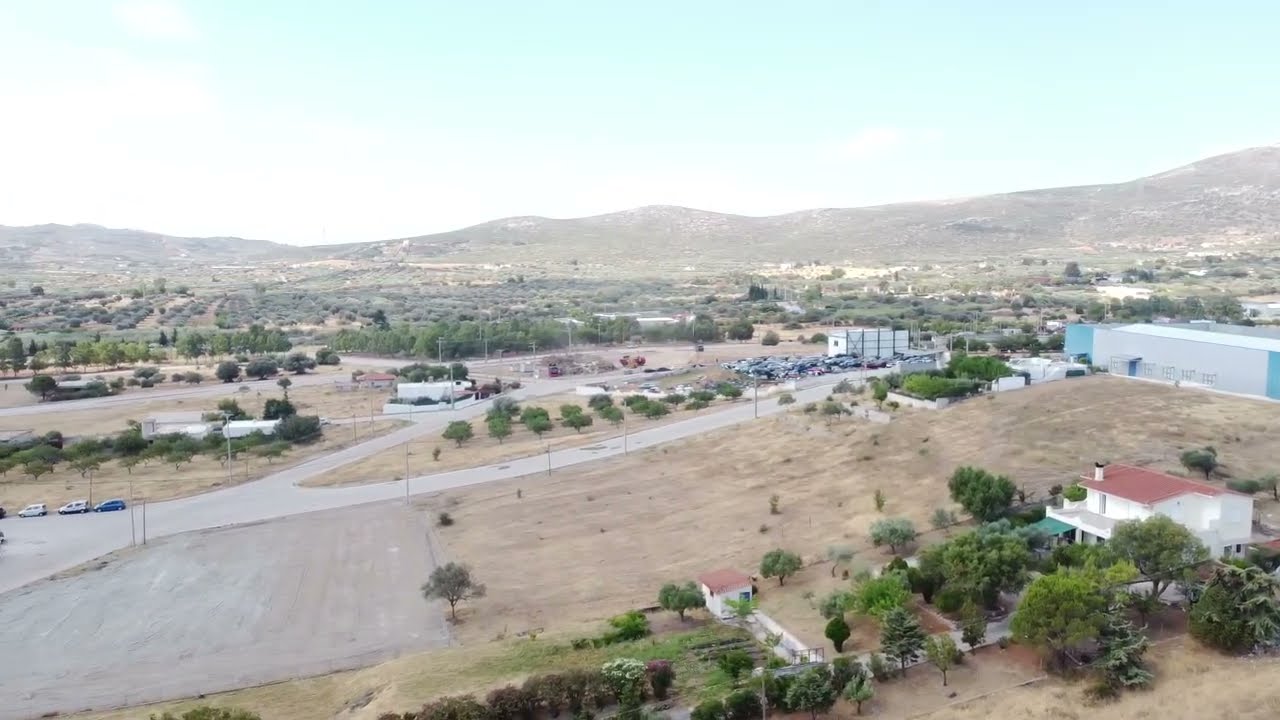This aerial photograph captures the outskirts of a town nestled against a mountain range under a clear blue sky. At the forefront, a picturesque white house with a distinctive red, possibly tin or brick-looking roof and a chimney stands prominently amidst some well-maintained landscaping. Surrounding the house are a few outbuildings, and behind it, a blue and white warehouse suggests some industrial activity, potentially a shipping or salvage yard.

The terrain around the house appears dry, hinting at a drought-like condition, with grass showing a yellowish-brown hue while the trees retain their green leaves. The community expands with various homes, businesses, parked cars, and a field, giving it a sense of a somewhat barren desert community. The mountains in the background provide a green contrast, growing progressively taller from left to right, enhancing the depth of the landscape. The intricate network of roads and a visible stoplight indicate nearby infrastructure, possibly an interstate. Earth tones dominate this elegant, wide-screen aerial photograph, highlighting the harmonious yet rugged beauty of this western townscape.